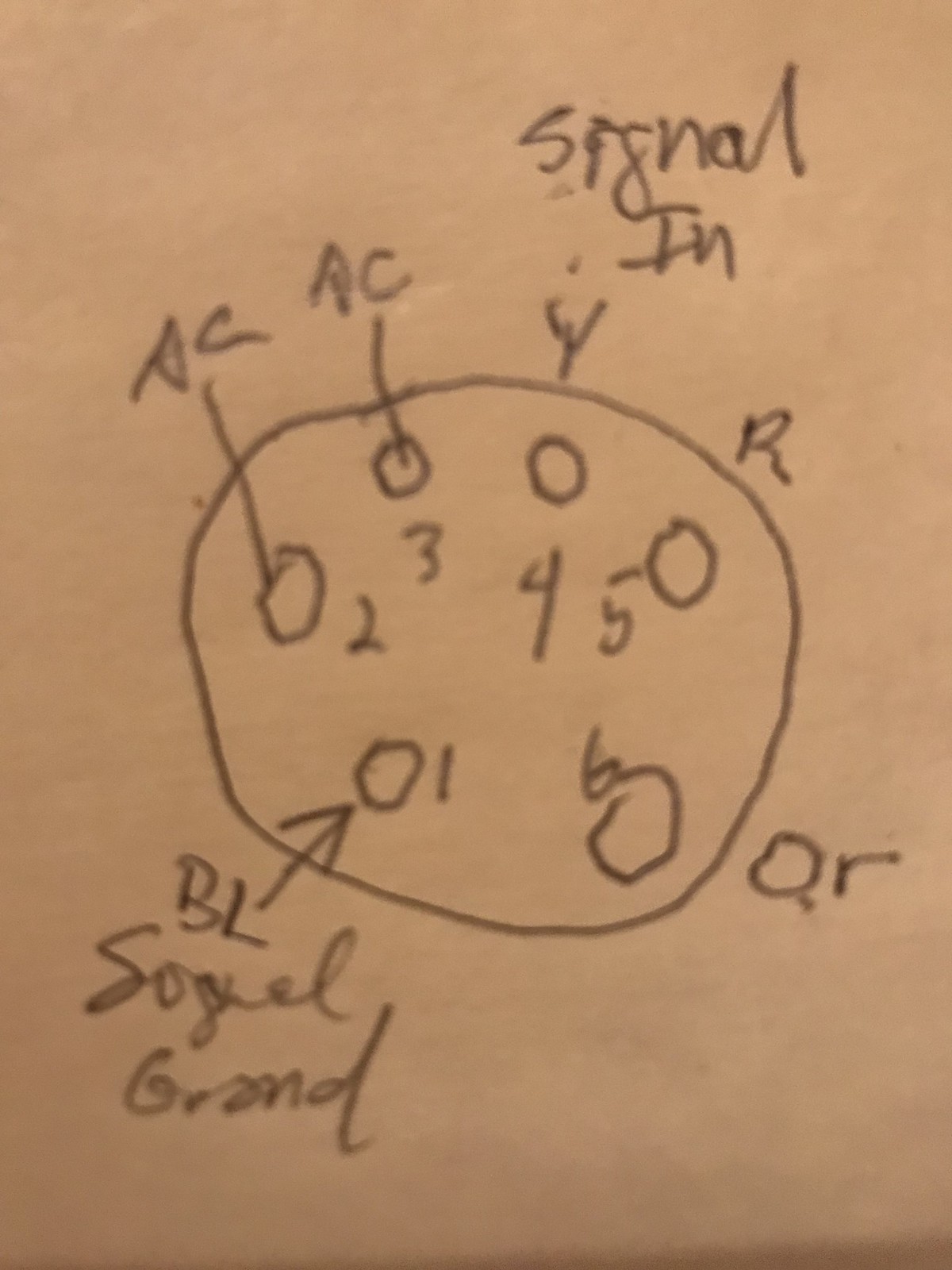The image features a close-up shot of a brown sheet of paper that resembles parchment but is actually regular brown paper. Drawn on the paper is a large, roughly sketched circle. Within this large circle, there are six smaller circles, each sequentially labeled from 1 to 6. These smaller circles have additional labels: Circle 1 is marked with an arrow and labeled "BL Sugarl Grand," Circle 2 and Circle 3 are both labeled "AC," Circle 4 is noted as "Signal N," Circle 5 is labeled "R," and Circle 6 is labeled "OR." The drawing appears hand-drawn and the labeling is clearly legible, indicating a schematic or diagram for reference purposes.